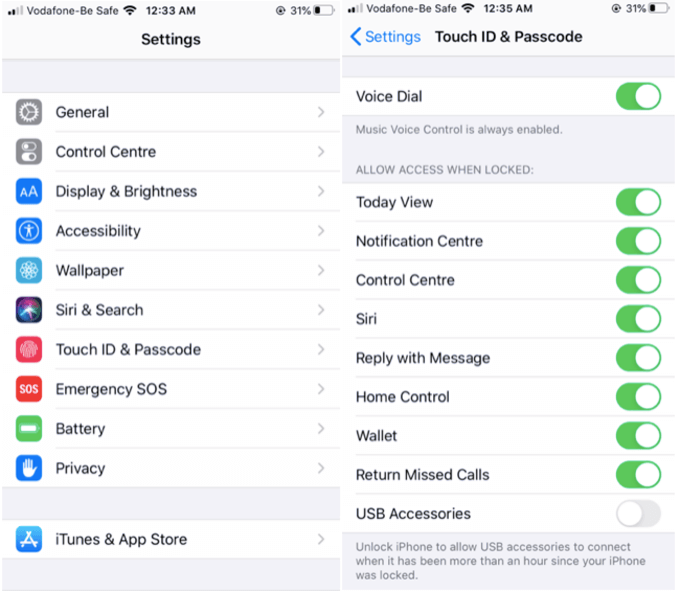The image displays two screens from a mobile phone device, showcasing different settings menus. On the left, the main settings interface is visible, containing higher-level settings categories: General, Control Center, Display & Brightness, Accessibility, Wallpaper, Siri & Search, Touch ID & Password, Emergency SOS, Battery, Privacy, and iTunes & App Store. The right side features a detailed view of the Touch ID & Password settings, which has been selected from the main settings menu. Notably, there is a time difference between the two screens: the clock reads 12:33 on the main settings screen and 12:35 on the Touch ID & Password settings screen, indicating a two-minute interval taken to navigate between these screens.

Within the Touch ID & Password settings, the following options are listed: Voice Dial, Today View, Communication Center, Control Center, Siri, Reply with Message, Home Control, Wallet, Return Missed Calls, and USB Accessories. All options are enabled, except for USB Accessories, which is disabled.